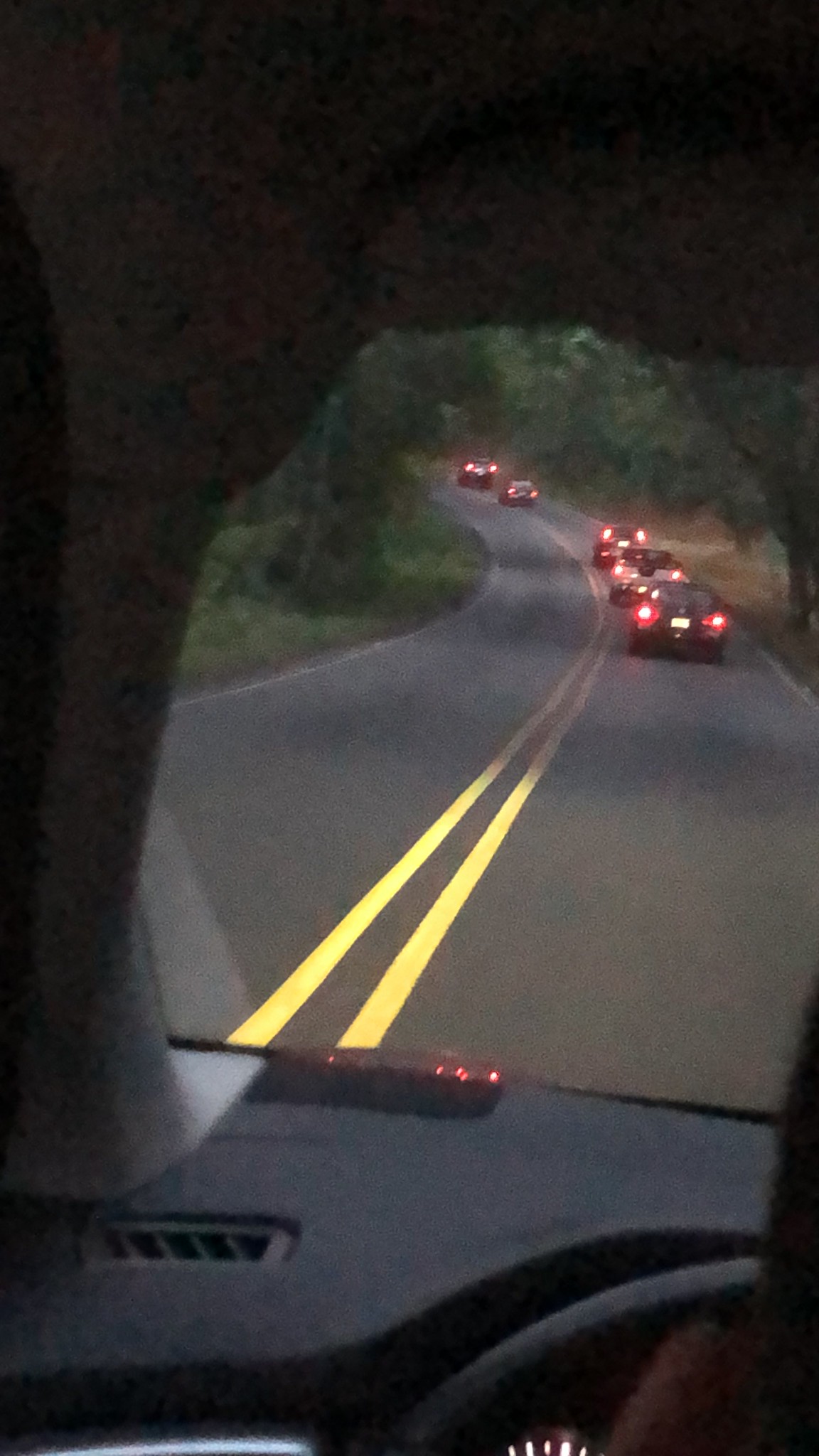In this low-resolution, vertically-oriented photograph, we view the scene from within a car, peering out through the windshield. The ambient lighting suggests it is either dawn or dusk, as the car’s headlights illuminate the dim surroundings and the tail lights of five cars ahead glow brightly. All the vehicles have emerged from a small tunnel with curved edges, indicating a single lane in each direction. The tunnel's exit frames the vehicles driving forward on the road. On the left side of the image, a vague and shadowed outline hints at the possible presence of a head, likely the silhouette of another passenger or the driver. The overall scene evokes a sense of early or late hours on a journey, transitioning from the confined tunnel space to the open road ahead.